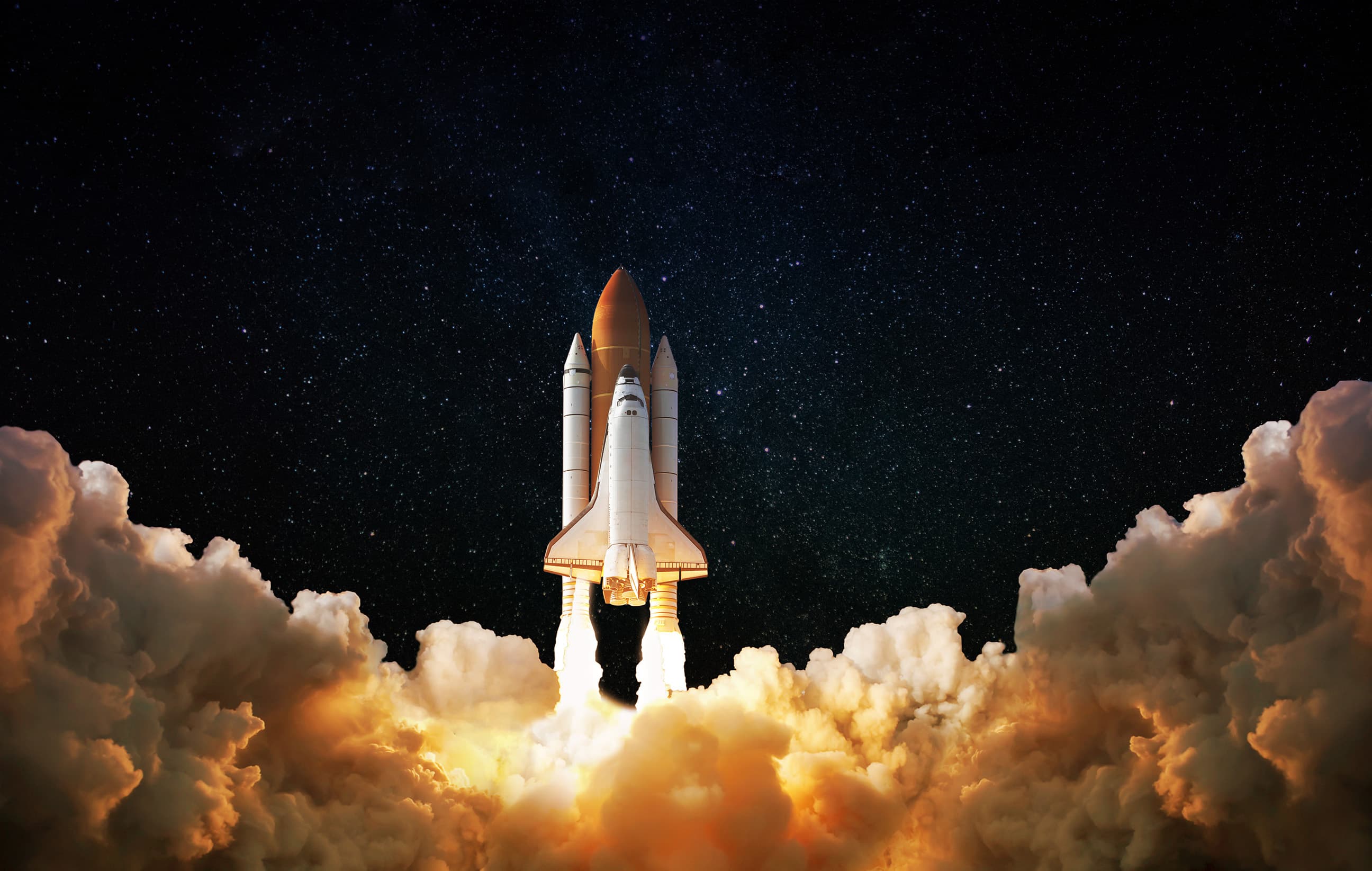This photograph captures a breathtaking nocturnal launch of a space shuttle. The central focus is the rocket, consisting of a prominent reddish-orange central segment flanked by two slimmer white rocket boosters. Vivid plumes of flame and smoke billow from the rocket's engines, delivering a spectrum of colors—from intense reds and oranges at the base to shades of whiter, yellower, and grayer hues as the exhaust disperses. The powerful engines' effect is evident as bright sparks and smoke envelop the bottom third of the frame. The rocket's ascent into the night sky is framed against a backdrop of a deeply black night peppered with countless stars. The scene’s intense contrast between the bright rocket and the starry night emphasizes the raw power and majesty of space exploration. The image captures a pivotal moment, with part of the rocket already enshrouded in space, exhibiting a subtle glow at its aft end. This stark yet dynamic portrayal of a rocket launch, emphasizing the detailed plume and atmospheric transition, presents a visceral and captivating snapshot of human ingenuity.